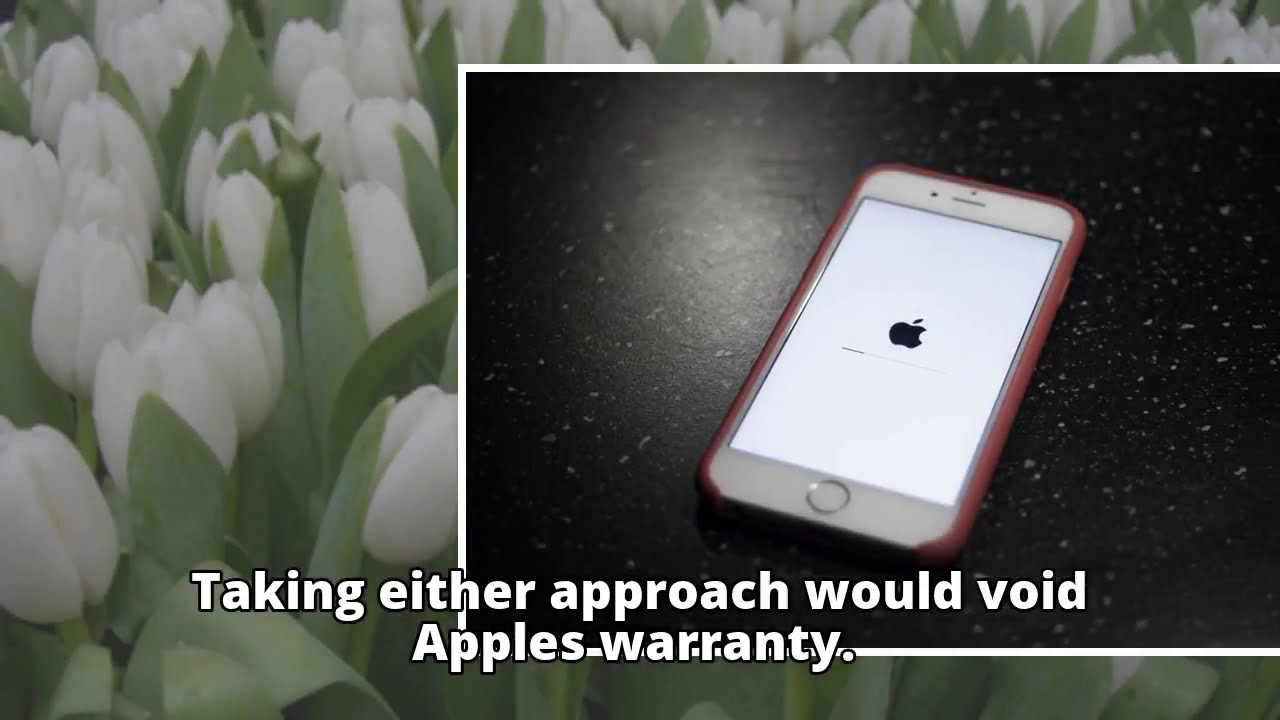In the photograph, a close-up of white tulips with lush green leaves forms the vibrant background, resembling a blooming field. The right side of the image features a large black box with delicate white speckles, upon which a white iPhone rests. The iPhone, appearing to be an older model due to its home button, is encased in a pink-toned cover, possibly salmon. The screen of the iPhone is on, displaying a prominent black Apple logo against a white background, suggesting it is in the process of restarting. Situated below the phone, in large white letters, a caption reads, "Taking either approach would void Apple's warranty." This striking visual juxtaposition highlights the serene beauty of the flowers against the modern technology set on a sleek black tabletop.